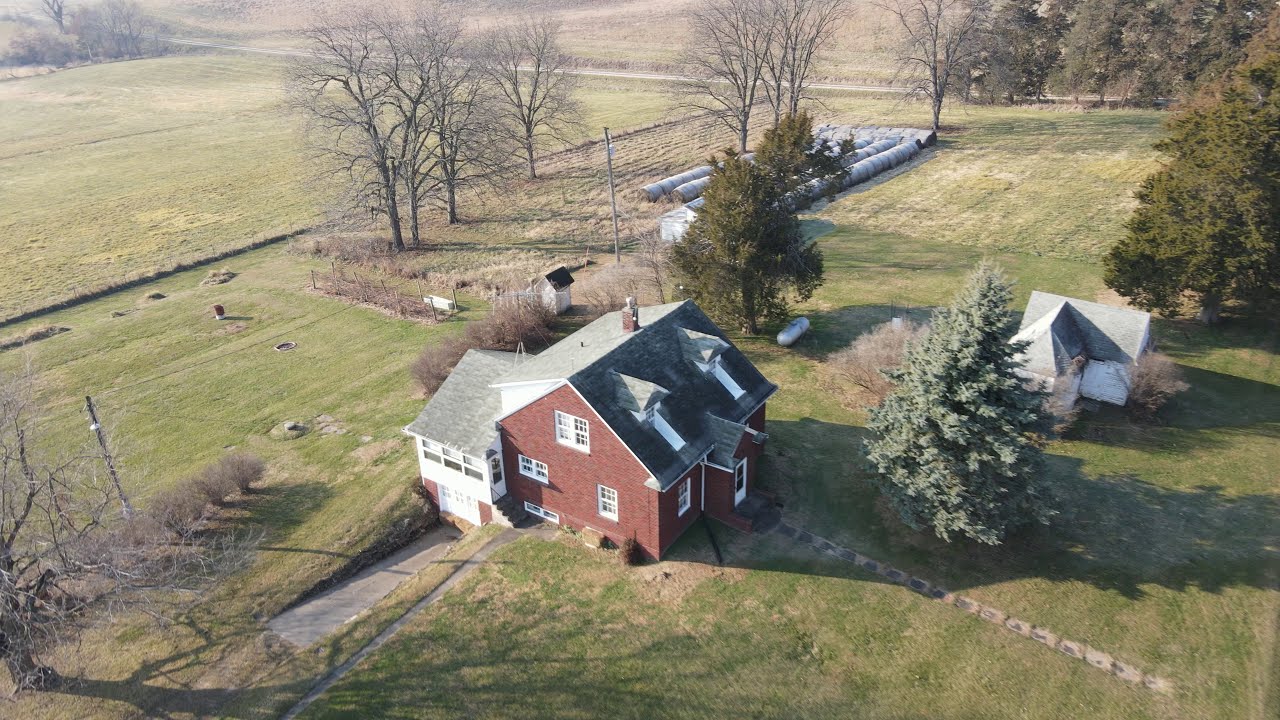An aerial photograph showcases a picturesque rural landscape, seemingly captured from a drone or aircraft, overlooking a vast field of mostly green grass, sprinkled with some brown patches indicative of late fall, winter, or early spring. At the heart of the image lies a charming two-story brick house with a gray roof and a central chimney. Attached to it is a white annex, with a driveway leading to the side. Nestled among the greenery, the scene features both bare deciduous trees and lush evergreens, adding texture to the flat terrain. Dominating the forefront is a monumental Christmas-like tree, accompanied by another large tree, framing the house beautifully. In proximity to the main house, there is a smaller white shed or guest quarters. Scattered throughout the field and bordering the landscape are more trees, some leafless, accentuating the season's transitional phase. A distant two-lane roadway hints at connectivity amidst this serene expanse, and off to the left, a solitary person appears to be standing, dwarfed by the vastness of the land around them.